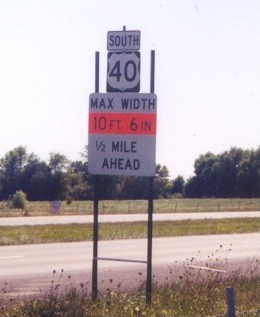The image features a road sign for U.S. Highway 40 South, indicating a narrowing road ahead with a maximum width of 10 feet 6 inches, within a half mile. The road is divided by a grassy median, suggesting it is summertime as the grass appears to be in need of growth. The scene is brightly lit with a pale blue sky overhead, although the sun is not visible. In the distance, trees border the road, adding a touch of nature to the setting. Additionally, a fence runs parallel to the road. The sign serves as a vital warning, especially for truckers, about the upcoming narrow passage on this otherwise typical roadway.